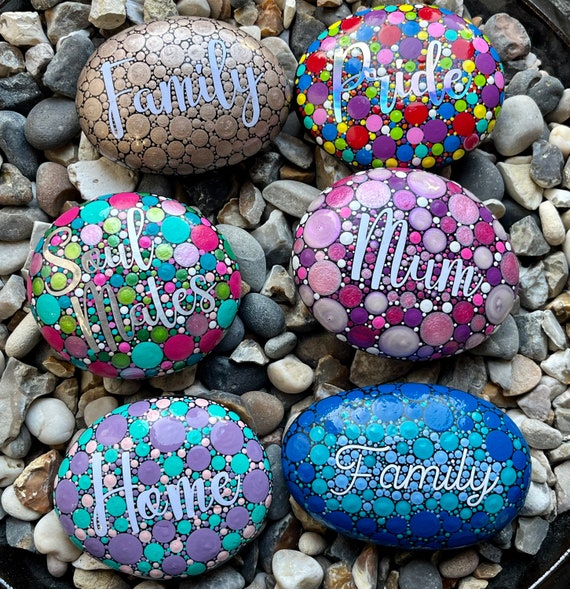This vibrant and artsy photograph showcases six intricately painted pebbles, each adorned with colorful designs and meaningful text. Arranged in three neat rows of two, the pebbles stand out against a backdrop of green rocks. In the top left corner, the first pebble is brown with round beige designs and the word "family" beautifully scripted in white. Next, a pebble featuring rainbow-colored circular patterns displays the word "pride." The third pebble, decorated with a multicolored palette of blue, green, pink, and red polka dots, carries the words "soul mates." The fourth pebble, in shades of lavender and pink, spells out "mum" in a distinctly British spelling. Following that, a pebble adorned with purple, blue, and white hues reads "home." Lastly, the sixth pebble, in varying shades of blue, also bears the word "family." Each stone's smooth, circular surface and meticulously painted backgrounds amplify the handcrafted, heartfelt nature of the artwork.